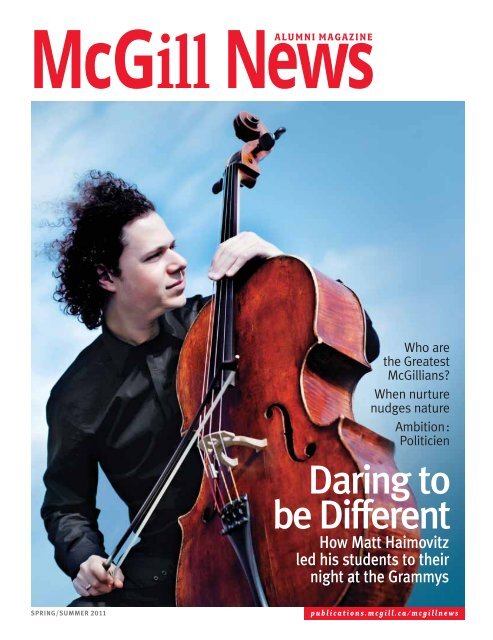The image is a vibrant magazine cover of the "McGill News Alumni Magazine," likely from Spring/Summer 2018. Dominating the cover is a striking photograph of a Caucasian man with long black curly hair, passionately playing a reddish-brown cello. He wears a black dress shirt and exudes intense concentration, his face stoic as he immerses himself in the music. The backdrop is a serene blue sky with clouds and light rays adding a dramatic effect as if he is playing outdoors. Surrounding his image are various textual elements: in bold white text on the left, it reads "Daring to be different: How Matt Helmuth led his students to their night at the Grammys," indicating his remarkable achievements in music education. Additional text on the right side ponders, "Who are the greatest McGillians? When nurture nudges nature. Ambition: politician," hinting at notable features within the magazine.